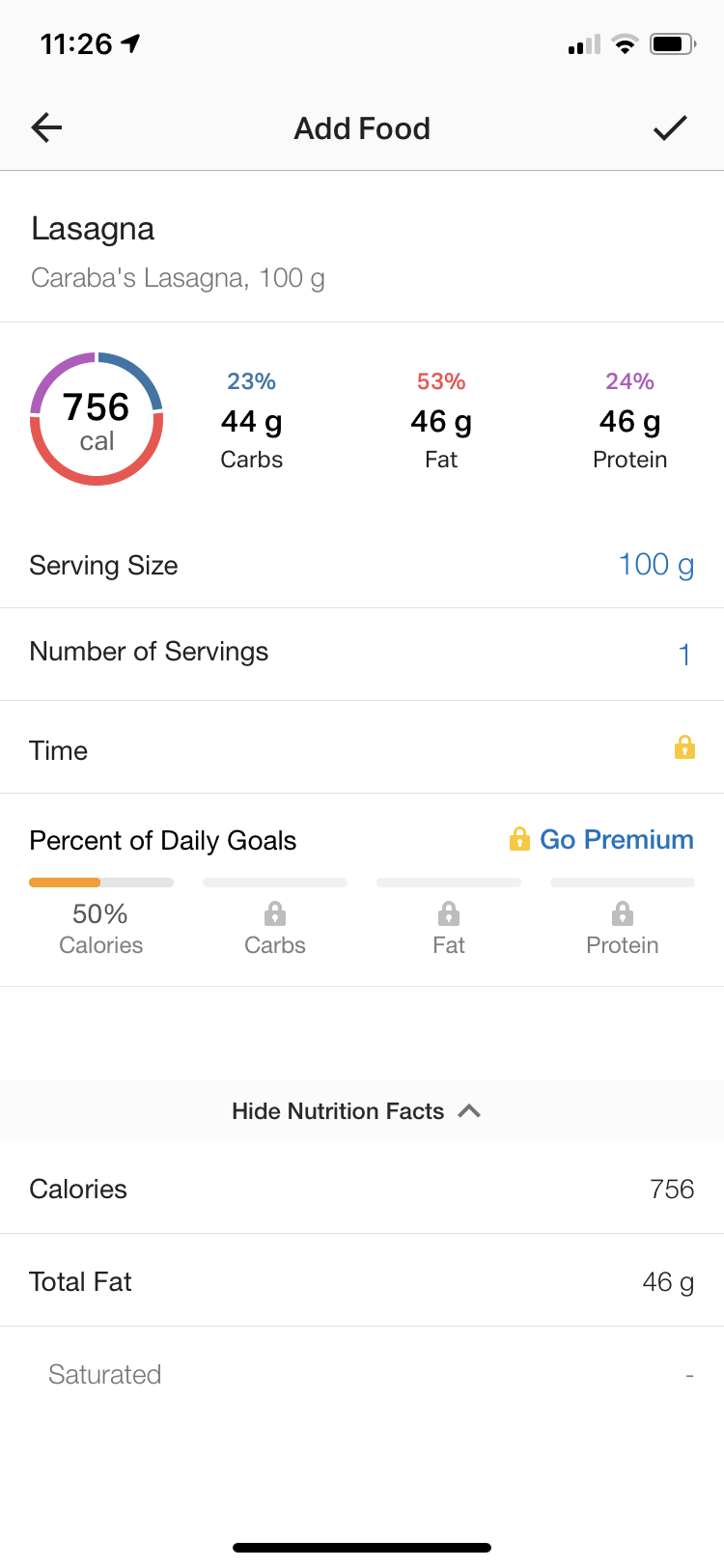A screenshot from a cell phone displays a page from a dieting or nutrition app. The time in the upper left-hand corner reads 11:26, while the upper right-hand corner shows two bars of cell phone signal strength, a Wi-Fi icon, and a battery icon. In the center of the top section, the text "Add Food" is prominently displayed, flanked by a left-facing arrow on the left side and a check mark on the right.

Below this header, the text "Lasagna" appears, followed by "Carrabba's Lasagna 100g." Further down, a multi-colored circle, consisting of blue, red, and purple sections, indicates that the lasagna contains 756 calories. The nutritional breakdown of the lasagna is detailed within the circle: 23% carbs (44g), 53% fat (46g), and 24% protein (46g).

The section following the circle lists the serving size as "100g" and the number of servings as "1." To the right of this section, next to the word "Time," there is a yellow lock icon.